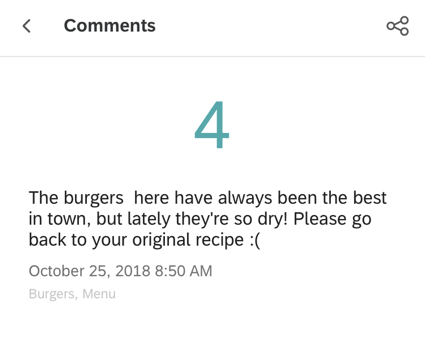In this cropped screenshot, likely from a Chrome or Android device given the presence of a distinctive network icon on the right-hand side not common to iPhones, the interface displays a comment section. At the top, a header labeled "Comments" is situated next to a left-pointing arrow icon for returning to the previous menu. Prominently, a large teal-colored number "4" is displayed, though it’s unclear whether this represents the number of comments or a rating.

Beneath the header, a user comment is visible: "The burgers  have always been the best in town, but lately, they're so dry! Please go back to your original recipe :(". This comment was posted on October 25th, 2018, at 8:50 a.m., and it raises curiosity about why someone would be commenting on burgers so early in the morning. The comment is tagged with "burgers" and "menu".

The comment section is on a white background with the header separated from the comments by a thin gray line. Additional informations, such as the date and tags, are displayed in light gray, while the comment text itself is in dark gray, creating a clear contrast for readability.